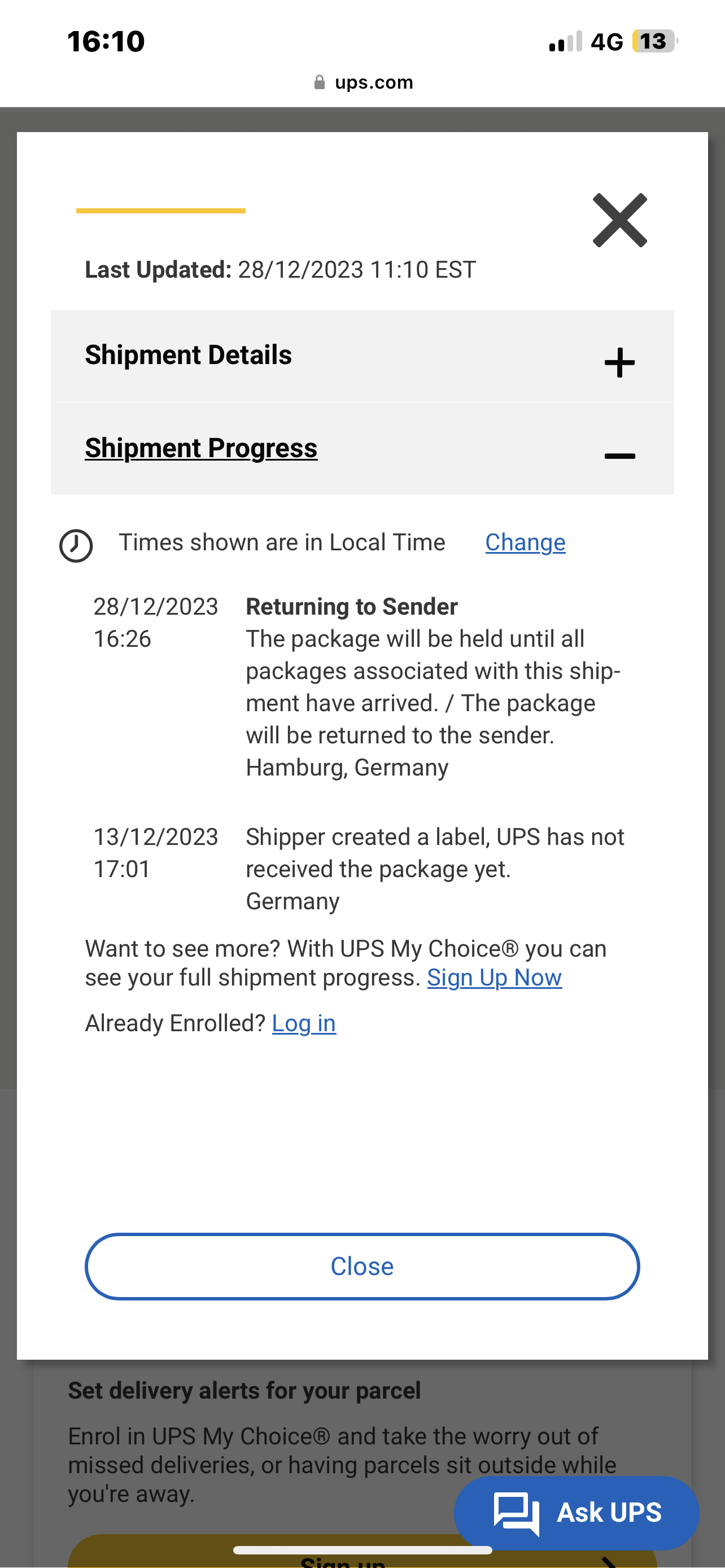This image displays a smartphone screen showing detailed information about an ongoing UPS shipment. The interface indicates a shipment status update and offers options for user interaction.

The upper portion of the screen has a white background. On the top left, the time is displayed as "16:10" in dark text. Centered directly beneath this, there is a small lock icon, and "UPS.com" is displayed. On the right side of the top line, indicators show 2 out of 4 bars for signal strength, "4G," and a battery level at 13%, represented by a number "13" and a battery icon.

The primary focus of the screen is a tall gray-outlined rectangular pane, taller than it is wide, with a grayed-out background. Over this, a white pane is superimposed, highlighted by a gray "X" on the top right, providing a way to close it. Directly beneath this, it states, "Last updated 28/12/2023 11:10 EST" in the same line.

Immediately below, a gray panel presents two lines of text:
- "Shipment details" followed by a plus sign (+)
- "Shipment progress" which is underlined, followed by a minus sign (-)

The information below the gray panel shifts to a white background, detailing the shipment's status updates:
- A header informs that "times are shown in local time" with the word "change" underlined in blue for altering display settings.
- The first entry, dated "28/12/2023," states, "Returning to sender at 16:26. The package will be held until all packages associated with this shipment have arrived. Package will be returned to the sender, Hamburg, Germany."
- The next entry, dated "13/12/2023 17:01," notes, "Shipper created a label. UPS has not received the package yet. Germany."

Further down, promotional text reads:
- "Want to see more? With UPS My Choice, you can see your full shipment progress." with "Sign up now" in blue and underlined.
- "Already enrolled?" followed by an underlined blue link to "Login."
- A white button outlined in blue in the center of the screen reads "Close" in blue text.

Finally, the bottom of the grayed-out original screen is faintly visible, encouraging users to "set delivery alerts on your parcel. Enroll in UPS My Choice and take the worry out of missed deliveries or having parcels sitting outside while you're away."